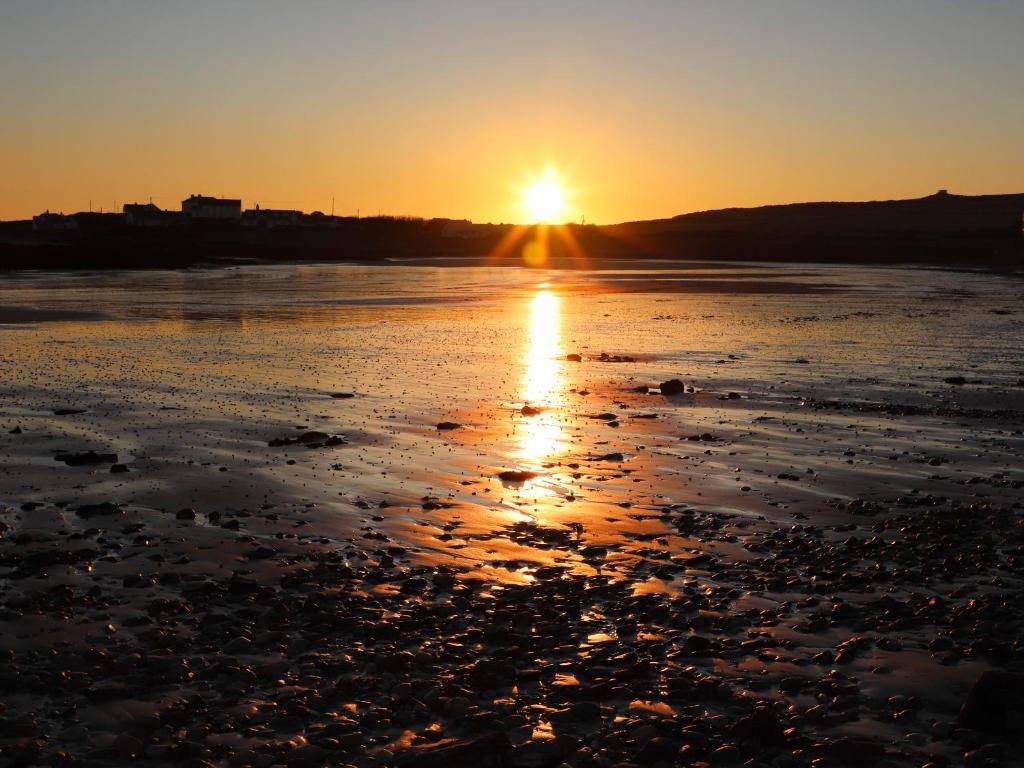This image captures a breathtaking sunrise (or possibly sunset) scene, with the sun either rising or setting behind a rugged, hilly mountain range. The glowing orb is positioned near the center of the sky, casting vibrant hues of orange and yellow that gradually transition to a darker blue as they extend upwards. The sunlight creates a striking reflection on the body of water below, forming a near-perfect mirror image.

The landscape beneath the scenic sky is enveloped in shadow, rendered in dark silhouettes. Scattered across the uneven, seemingly messy terrain are small, lumpy rocks and round items, possibly sediments or textured elements, adding to the rugged appearance. This shadowed ground contrasts sharply with the bright, reflective lake or ocean, enhancing the visual impact of the scene.

On the left side of the image, a few small, square buildings—possibly houses or warehouses—are visible, emphasizing the human presence amidst the natural beauty. The reflective surface of the water or wet sand extends towards these structures, creating a dynamic interplay of light and dark.

The overall composition, with its vibrant sky, reflective waters, shadowed landscape, and scattered buildings, evokes a sense of serene beauty combined with a hint of rugged wilderness.